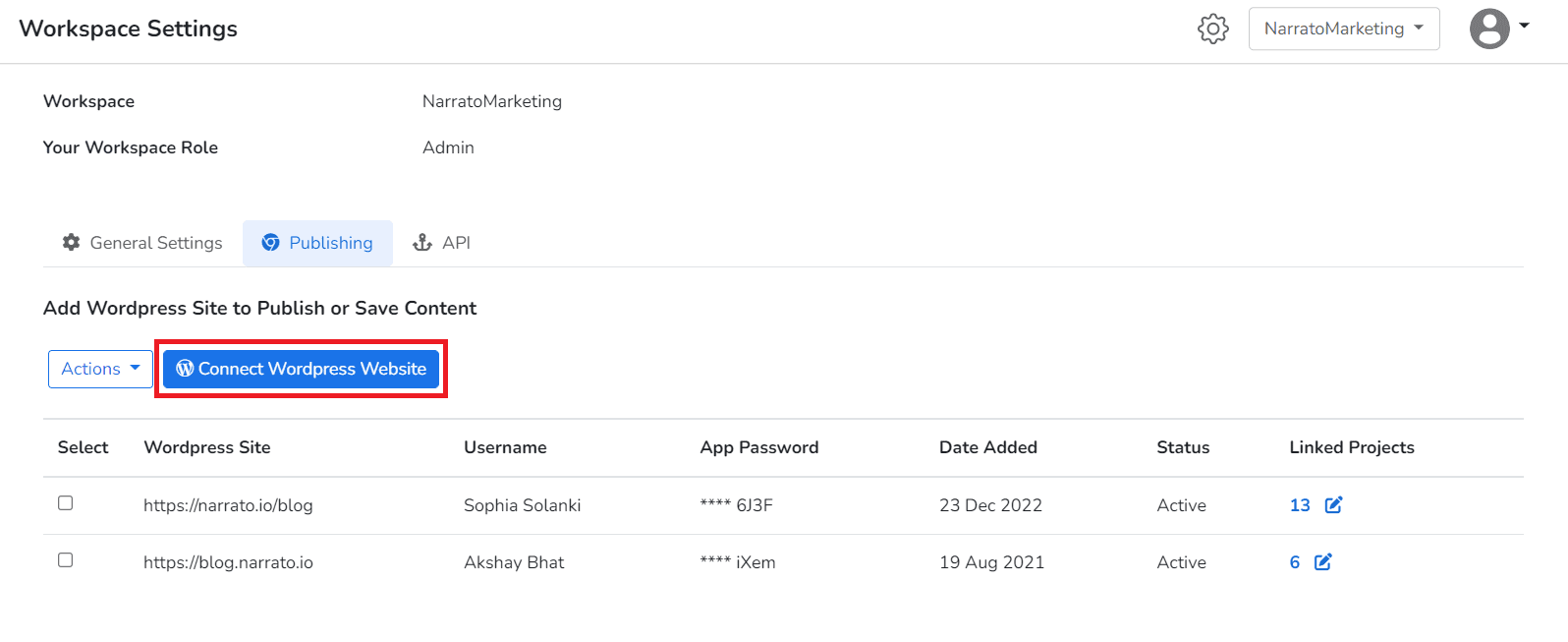In this color screenshot of the workspace settings for an application, the landscape-oriented image features a workspace titled "Nereito Marketing," with "N" and "M" both capitalized. The user viewing the settings has an admin role, indicating they possess the highest level of access within this workspace.

The interface is divided into three primary tabs: General Settings, Publishing, and API. The screenshot captures the moment when the user is on the Publishing tab. Under this tab, there is an option to "Add WordPress Site to Publish or Save Content," accompanied by a large, dark blue button labeled "Connect WordPress Website." This button is highlighted further by a dark red rectangle surrounding it, drawing significant attention.

Below this call-to-action button, the screenshot lists two connected WordPress sites: "harato.io/blog" and "blog.narato.io." The associated usernames for these sites are Sophia Selensky and Akshay Bhatt, respectively. Additionally, the display includes partial information concerning their passwords and the dates these sites were added to the workspace. This detailed setup provides an organized view of the current publishing configurations within the "Nereito Marketing" workspace.